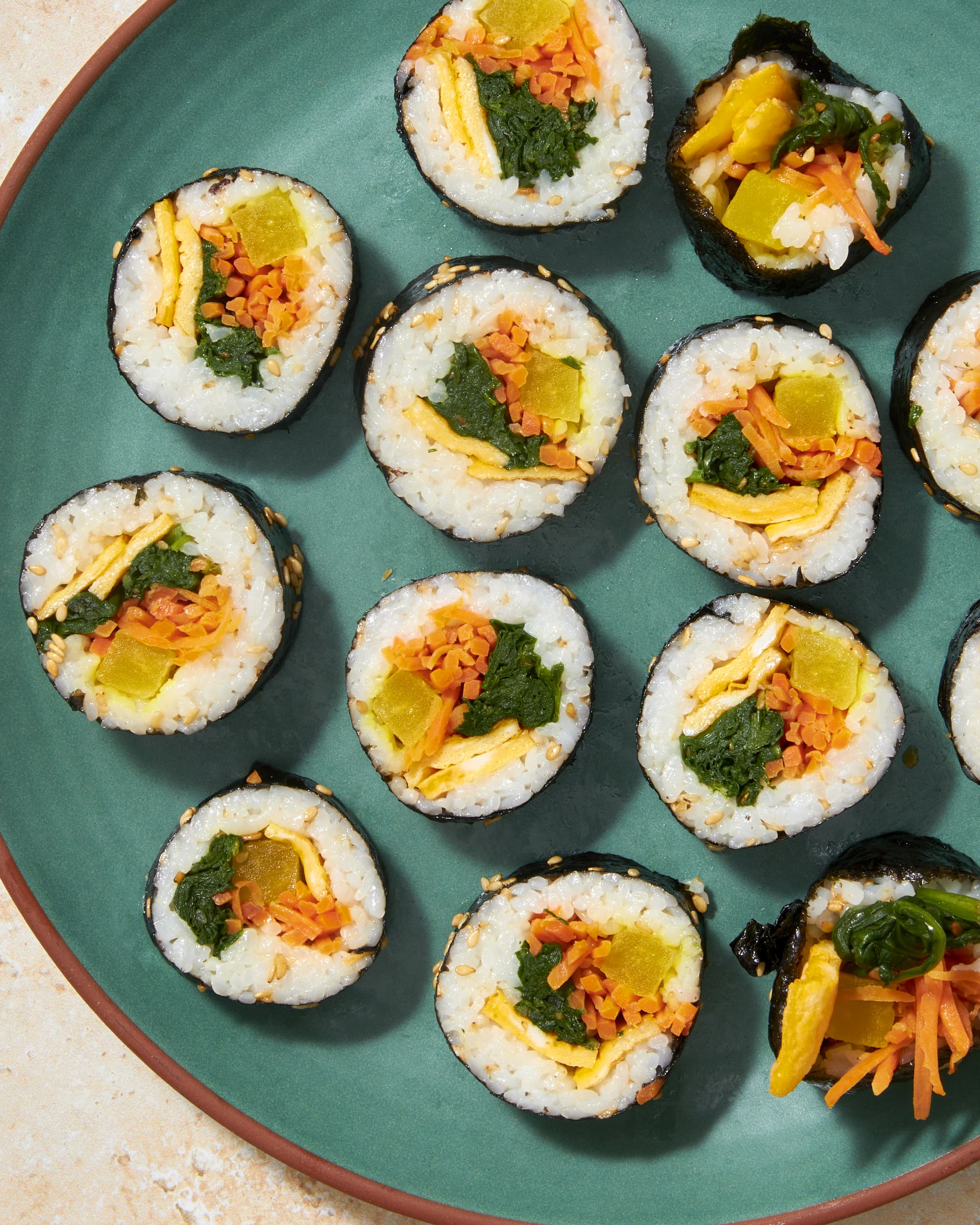This image captures a close-up, top-down view of a greenish-blue ceramic plate with a red border and ridged concentric circles, showcasing an assortment of sushi rolls. The variety of sushi, at least 14 pieces, includes some with yellow fish, brown rice, and green seaweed, all wrapped in black seaweed with white rice visible inside. The sushi pieces are meticulously arranged on the plate, except for one in the lower right corner that appears messily assembled with more prominent yellow, orange, and green ingredients. The plate itself, with its upward-curving edges, sits on a light tan, stucco-like table surface, which is partly visible at the corners of the image.